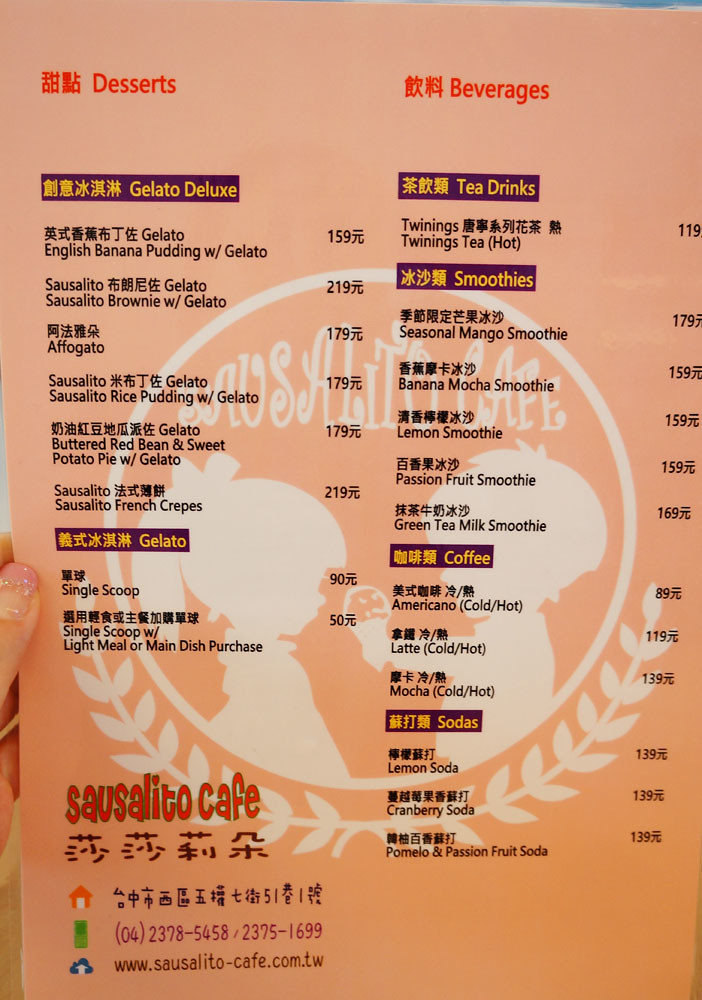A detailed close-up image of a pink menu reveals a well-manicured, polished thumb holding the menu up, partially visible near the center-left. The menu is predominantly written in both English and Chinese characters and is divided into two main sections.

On the left-hand side, under a red header labeled "Desserts" with adjacent Chinese characters, the menu lists various items:
- "Gelato Deluxe" in yellow on a dark border
  - Gelato
  - English Banana Pudding with Gelato priced at 159 units of an unspecified currency
  - Sausalito with Gelato
  - Affogato (with accompanying Chinese characters)
  - Rice Pudding with Gelato
  - Buttered Red Bean and Sweet Potato Pie with Gelato
  - French Crepes

A new section starts with another yellow-bordered header:
- Gelato
  - Single Scoop
  - Single Scoop with Light Meal or Main Dish Purchase (both in English and Chinese)

On the right-hand side, a red header similar to the left reads "Beverages" with Chinese characters next to it, listing categories such as tea drinks, smoothies, coffees, and sodas.

At the bottom left corner, "Sausalito Cafe" is written in red with Chinese characters beneath it, identifying it as a Taiwanese restaurant. Additional Chinese characters, a phone number, and a website are listed below, providing further contact details.